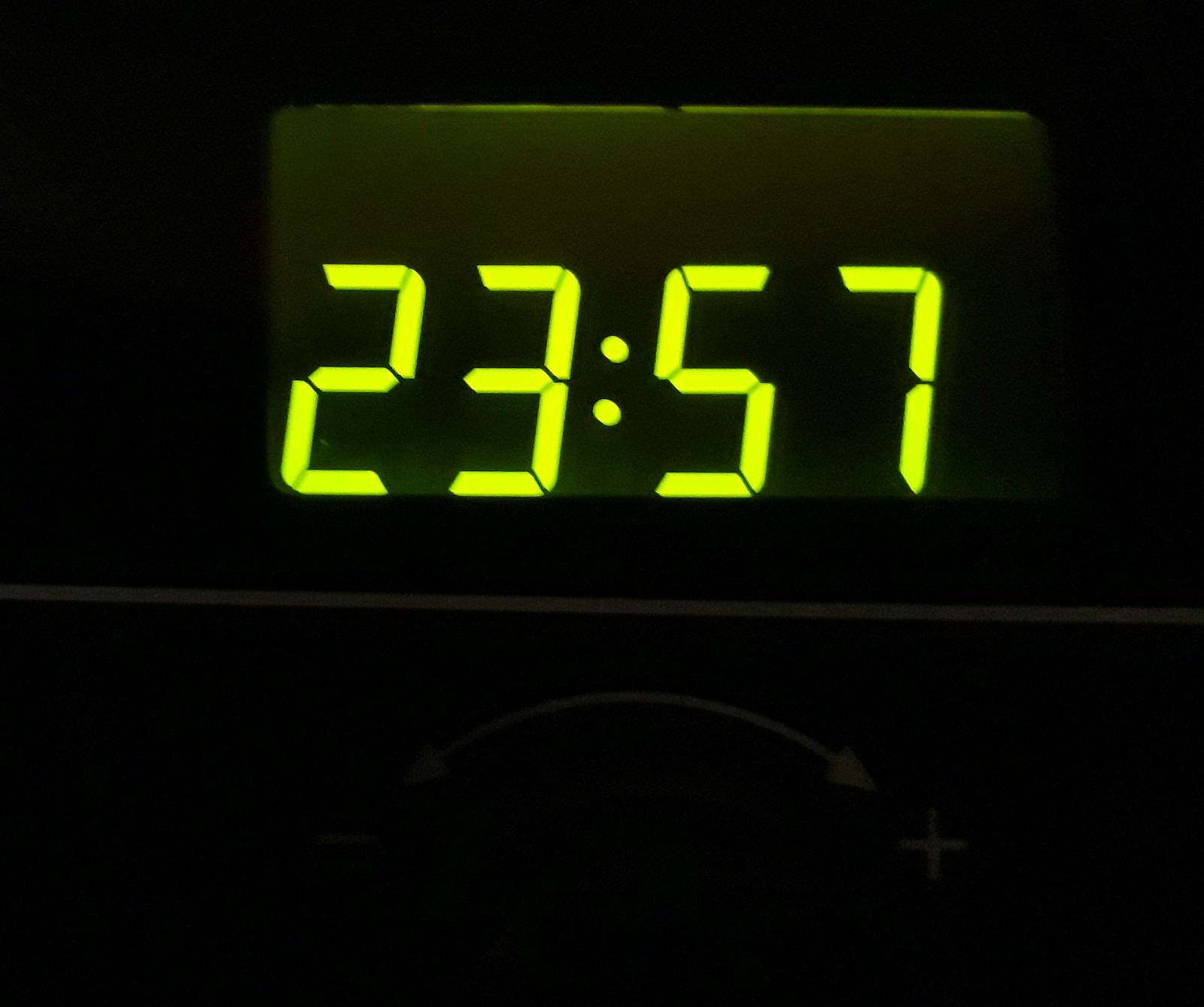A highly detailed close-up image of a digital clock with a black face. The screen of the clock has a green tint, displaying the numbers "23:57" in a bold, digital font. The clock's display area is divided by a horizontal white line running through the center of the image. Below this line, there is a semi-circular graphic with arrows on each end. The left arrow, pointing to a minus sign, and the right arrow, pointing to a plus sign, are all depicted in white.